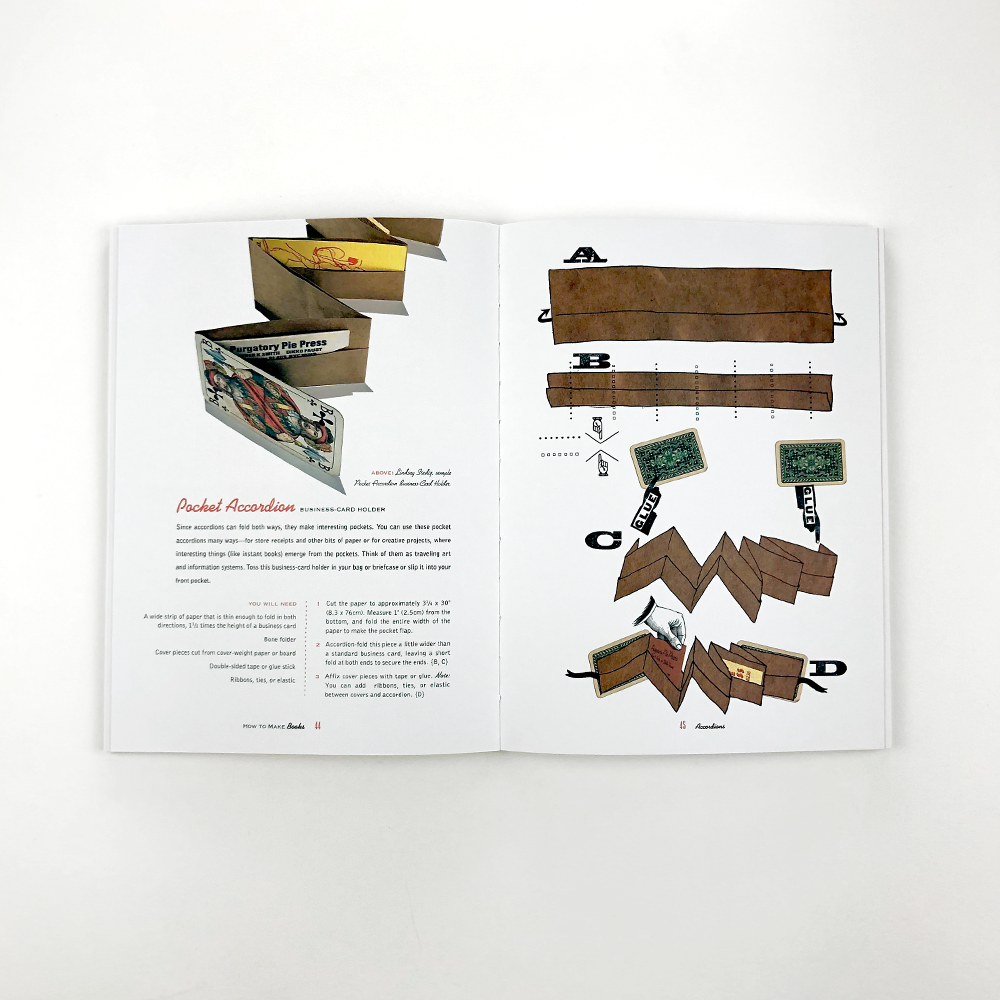The square-oriented image features an open book against a white to light-gray background. In the center of the image, the book displays two pages detailing how to create a pocket accordion business card holder. The left page shows an illustration of the finished product—a partially opened pocket accordion with a playing card affixed to its front. Beneath this, there is a paragraph of justified text followed by two columns of additional instructions. The right page features step-by-step illustrations labeled A, B, C, and D, demonstrating the construction process. A and B depict brown horizontal rectangles, with B being thinner than A. In the middle, two navy and white bordered playing cards are labeled with "glue." The lower sections C and D show the folding process of the brown paper into the accordion shape.